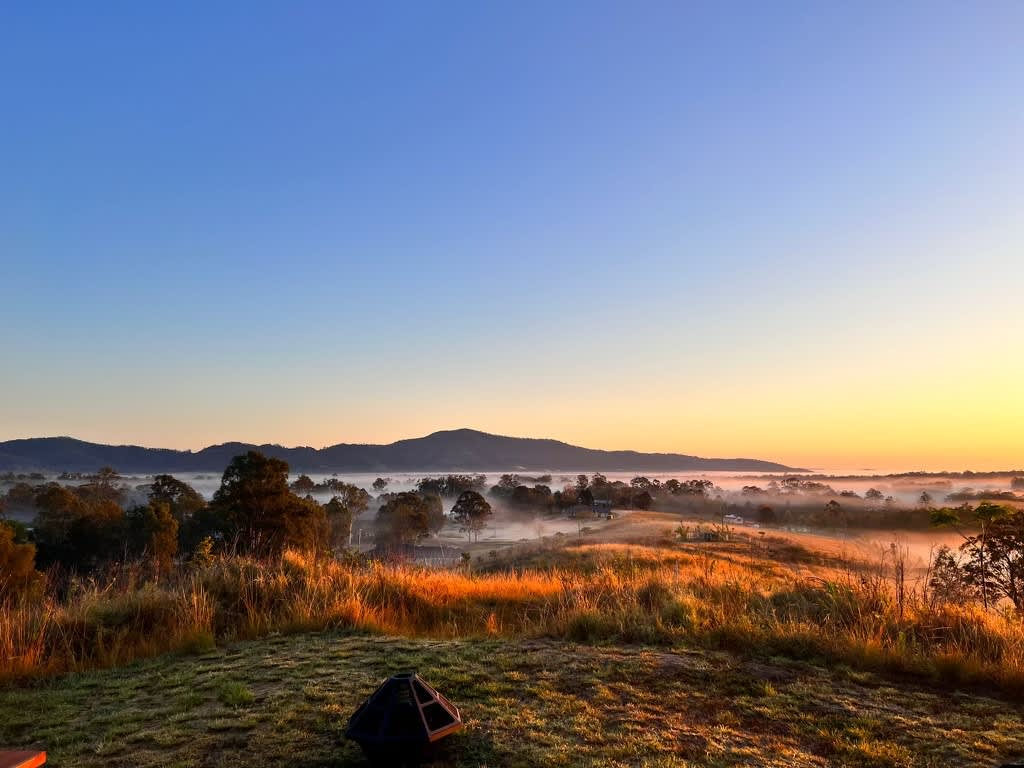The image captures a serene outdoor setting marked by a striking contrast between a vibrant sky and rich natural elements. The top half of the image shows a blue sky transitioning into a haze of yellow and orange hues towards the horizon, with some faint clouds creating an ethereal effect. Just below the sky lies a distant range of black mountains that become slightly lighter as they stretch across the image. Moving down from the mountains, an expanse of mist blankets a dense forest of dark green trees, creating a mystical ambiance. 

Beneath the tree line, various patches of wild, unkempt grass intermingle with more trampled, brown-tinged grass, leading towards the bottom of the image. Here, a closer inspection reveals distinctly green and brown patches of grass. The scene also includes a small, pyramid-shaped wooden structure in the center-bottom of the image, which is brown with some white and yellow highlighting its base. This tranquil landscape seems to reflect a morning setting, characterized by the golden light and the presence of fog. Scattered field weeds and hints of an underlying water body add layers of texture and depth to this picturesque scene.